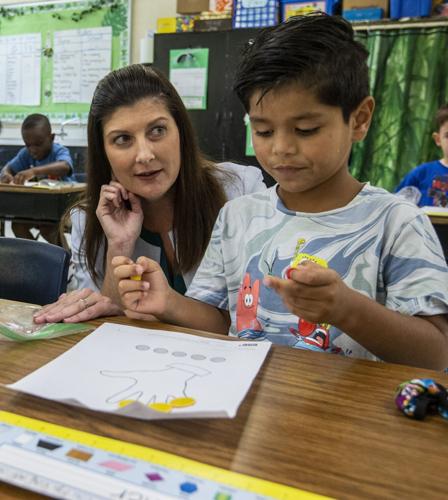In a bustling classroom, a young Hispanic boy, approximately four years old, sits at a light brown desk adorned with an Elmo T-shirt as he intensely concentrates on his activity. He appears to be placing yellow plastic coins or discs on the fingertips of a handprint in front of him, possibly finger painting. Beside him, a teacher with long brown hair, dressed in a light blue jacket, leans in with a half-smile, offering encouragement and guidance as she rests her hand on her face.

The background is filled with classroom materials and decorations: a board covered in papers with black text, a chalkboard, and a whiteboard, each displaying various classroom information. Over the teacher’s right shoulder, an African-American boy in a blue shirt works diligently on his own task. Another student, partially visible, wears a blue shirt with red writing.

Atop the boy’s desk, there is a yellow ruler and a sign decorated with multi-colored shapes, adding a vibrant touch to his workspace. An unidentified toy is also present. Behind the children, a green shower curtain presumably serves to conceal storage, while a cabinet holds lunch bags with a calendar featuring green artwork pinned to it. Two signs, possibly displaying class rules or birthdays, hang on the wall, completing this lively educational scene.